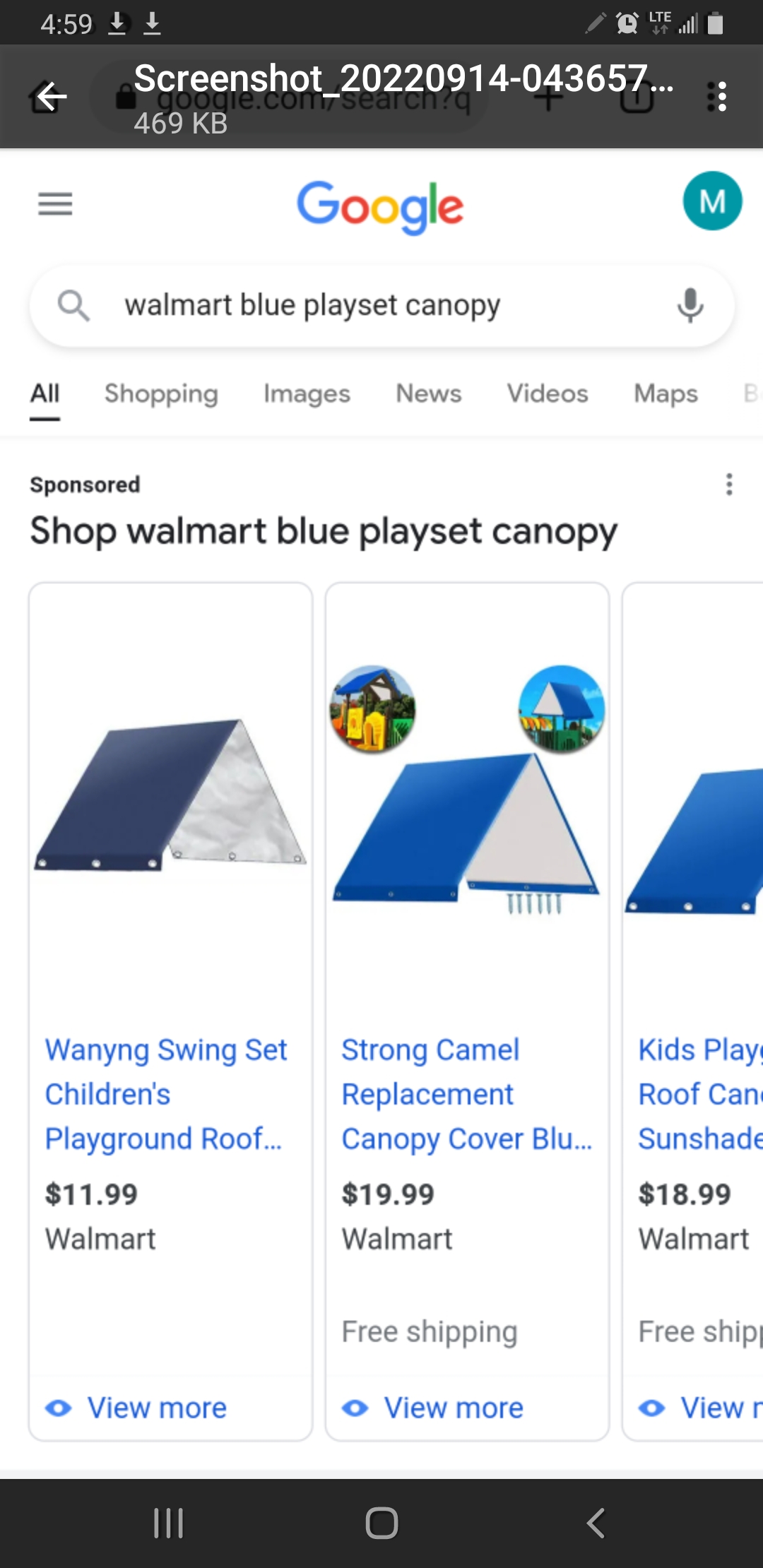The image is a screenshot taken from a mobile device, displaying the Google Chrome web browser. At the top of the image, there is a gray banner indicating the word "screenshot" along with the file size of 469 kilobytes. The screenshot captures a Google search results page for the query "Walmart blue playset canopy." 

Below the search bar, tabs for various search categories such as "All," "Shopping," "Images," "News," "Videos," and "Maps" are visible. The first visible result is a sponsored link advertising the "Walmart blue playset canopy." 

The search results begin with a product listed as a "Winning Swing Set Children's Playground Roof," priced at $11.99 at Walmart. The second item is described as a "Strong Camo Replacement Canopy Cover in Blue" for $20.99, also available at Walmart with free shipping. The third item, partially cut off, mentions a "Kids Playground Roof Canopy Sunshade" for $18.99 from Walmart.